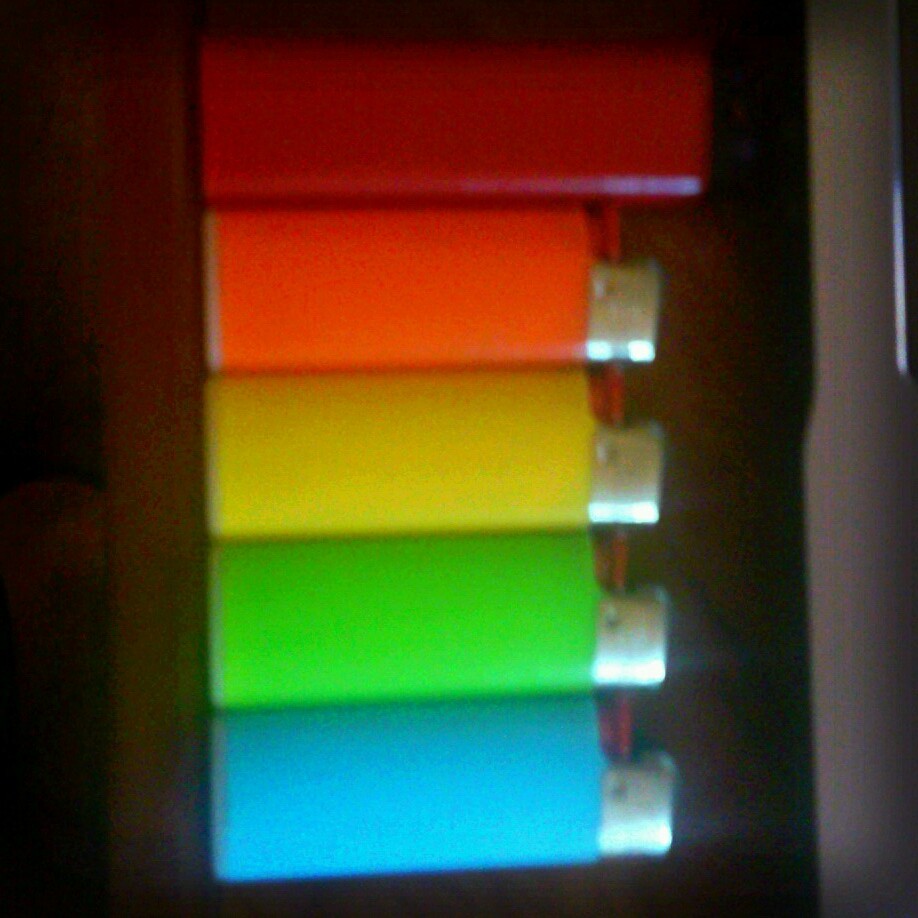This image depicts a blurry photograph of five objects resembling BIC lighters, arranged in a seemingly stacked manner against a brown background. From bottom to top, there is a baby blue lighter, followed by a green lighter, a yellow lighter, and an orange lighter. Each of these lighters features a silver top and a red ignition button, typical of classic plastic lighters. At the top of the 'stack' is a slightly longer, solid red object with a black top, which resembles a lighter but is distinct in its size and color. The lighters are brightly colored, evoking a sense of primary, vivid hues. There is a gray line on the right side of the image and a black section towards the left, possibly indicating other objects or parts of the setting, though the image's overall blurriness makes it hard to determine their exact nature. The orientation of the lighters and surroundings might suggest they are either laying flat or inside some container, and the photograph might have been taken at an angle, creating the illusion of stacking.